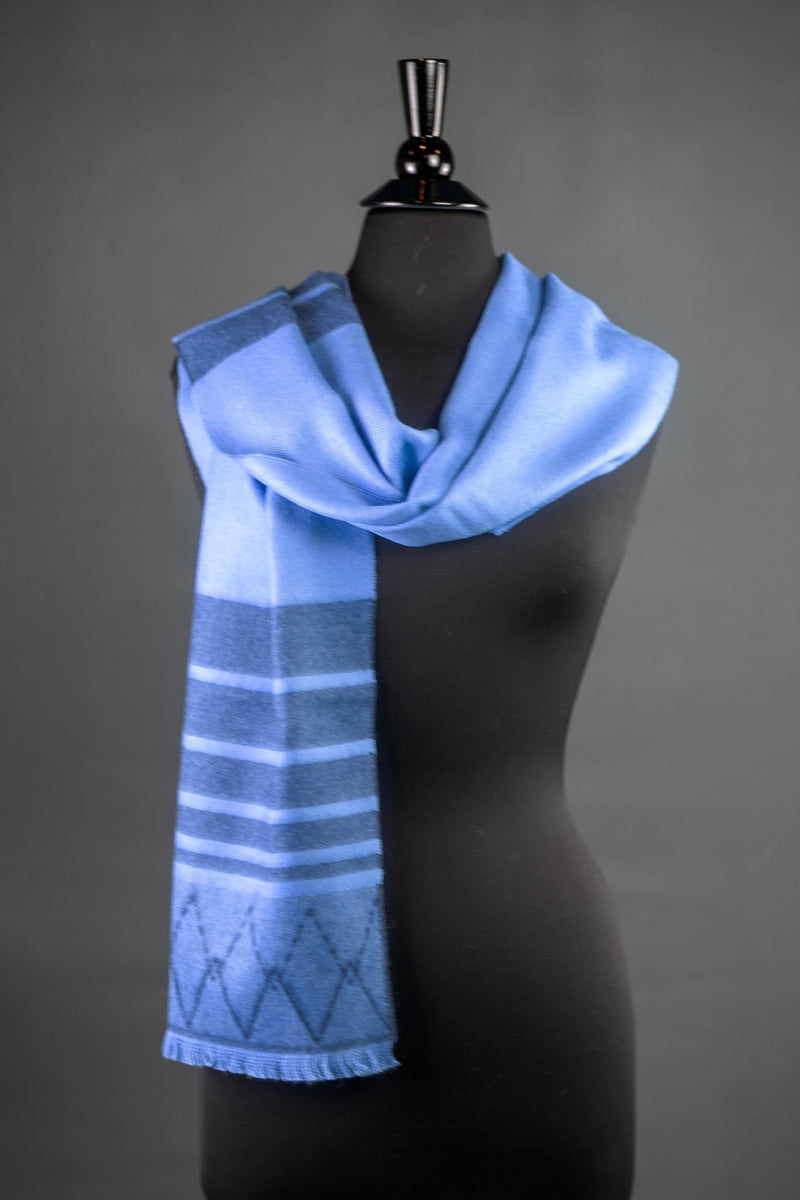The image depicts a matte black mannequin set against a charcoal gray background, primarily showcasing the torso, shoulders, and the upper parts of the legs, but notably missing arms and a complete head. At the top of the mannequin, where the head would be, there is a glossy black metallic structure consisting of a triangular base topped with a round piece, followed by a cylinder. Adorning the mannequin is a blue scarf, which exhibits various shades of blue, including light blue and darker blue patterns. The scarf is draped elegantly around the mannequin's neck, forming a loop on the chest with its left end hanging down to just below the waist, showcasing black horizontal bars and darker blue diamond shapes near the fringe. The right side of the scarf is thrown back, leaving the right shoulder exposed. The scarf’s end on the left features distinct segments that grow thinner towards the bottom, culminating in a thicker light blue segment adorned with blue diamond outlines, finishing with a blue fringe.